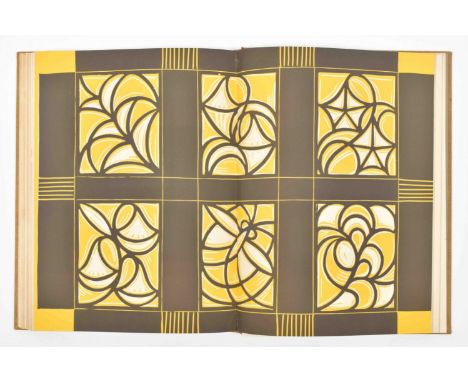This image depicts an open book with a detailed, symmetrical design spanning both pages. The book's cover is a brownish color, framing the central artistic display. The design is characterized by a grid-like pattern, divided into six distinct squares, each square containing unique, intricate yellow and white designs reminiscent of stained glass or floral motifs, bordered by dark gray lines. A decorative brown lattice, accentuated with yellow lines, separates the squares. Vertical gray stripes mark the edges and center of the pages, enhancing the appearance of a continuous and harmonious layout. The overall aesthetic suggests an art book, as there is no text, only a beautifully illustrated plaid-like pattern with floral and vine elements in shades of yellow and gray.